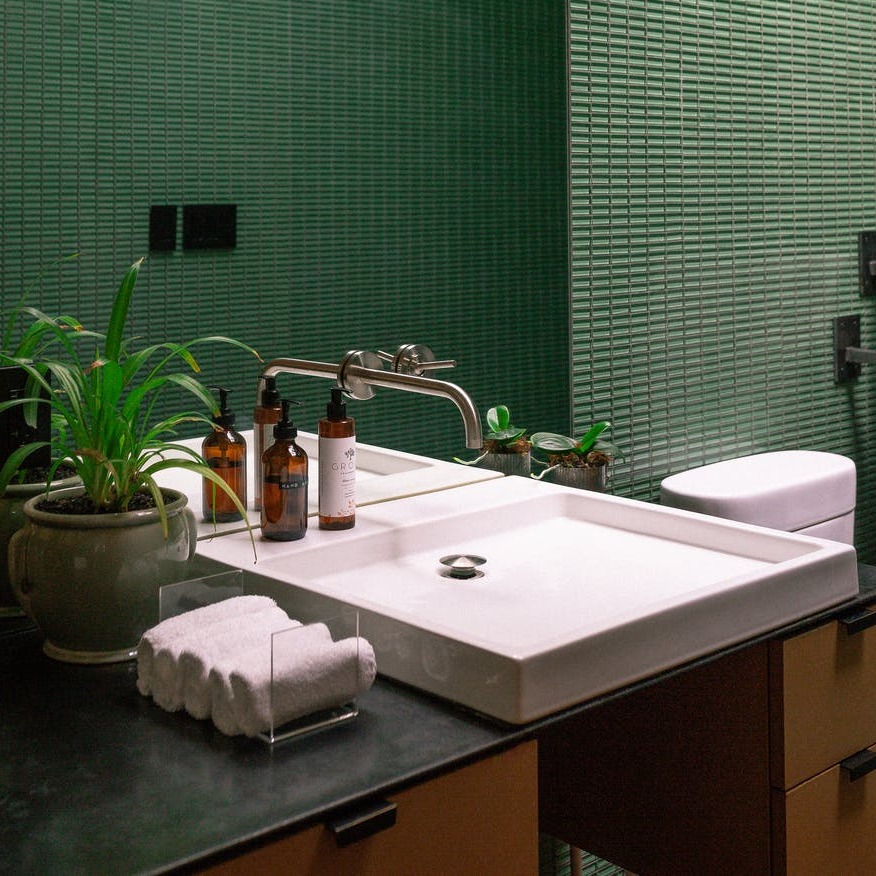This photograph captures a modern bathroom sink area with distinctive design elements. The image, shot from above, reveals a square white ceramic sink that is relatively shallow with a silver pop-up drain and a long stainless steel faucet protruding from the wall behind it. The wall itself serves as a mirror, reflecting the sink, a green plant, and the adjacent elements. Dark green tiles with raised rectangular patterns cover the walls around the basin, giving a textured look. 

On the left side of the black countertop, next to the sink, there is a potted green plant with side handles and a clear plastic container holding rolled white hand towels. Adjacent to these elements are two brown bottles, likely containing hand soap and lotion, sitting towards the back of the sink. Below the countertop, there are brown wooden drawers with black handles. Additionally, a silver knob is visible to the right of the faucet, and a black electrical outlet is mounted on the wall. The consistent reflection in the mirror showcases the cohesive, modern aesthetic of the bathroom design.